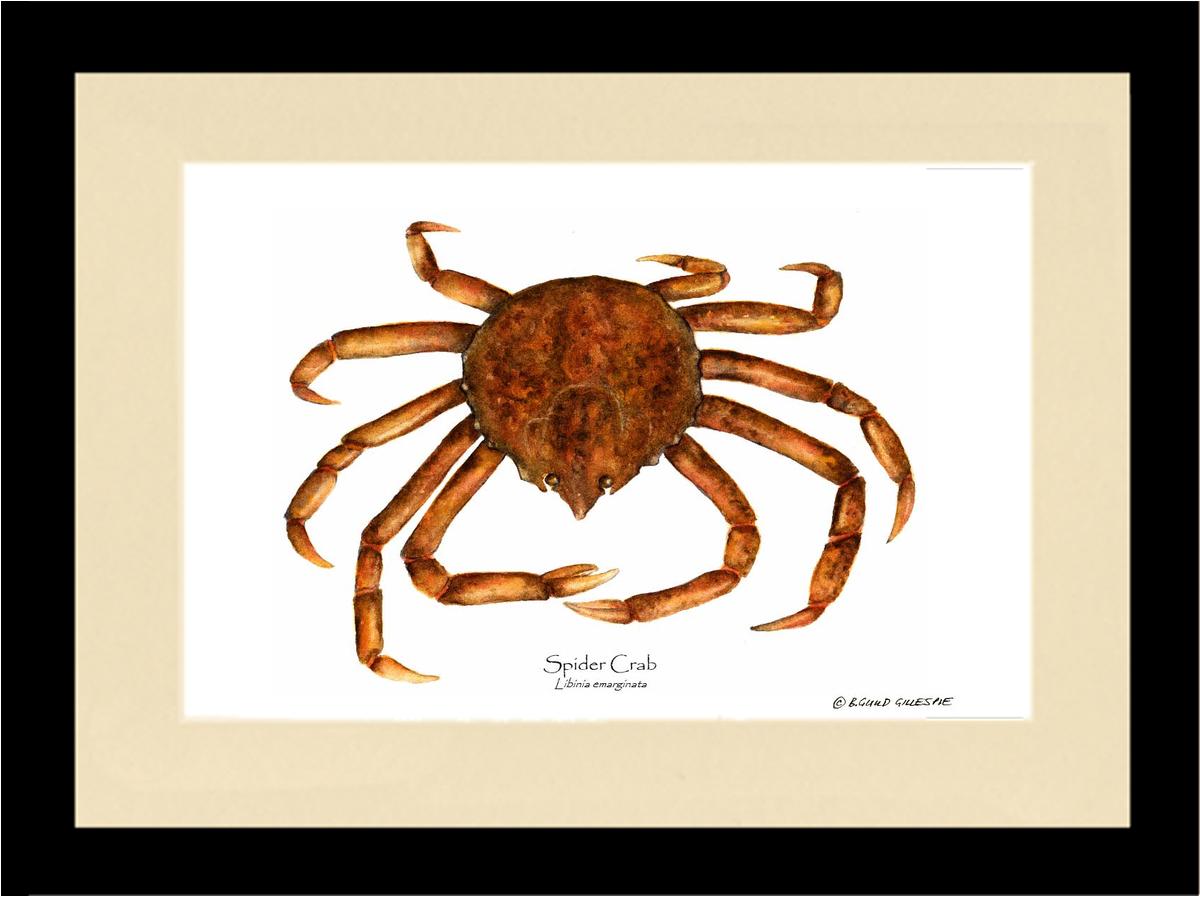The image is a detailed drawing of a large brown-orange spider crab, centrally framed and occupying roughly half of the overall space. The crab, identified by the text "Spider Crab" near its bottom center, features a darker brown mottled shell and lighter-colored legs, ten in total, five on each side. Beneath its depiction, the Latin name "Labinia Emarginata" is inscribed. The crab has small claws at the tip of each leg and two small, noticeable brown eyes. The artwork is surrounded by an oatmeal-colored mat and encased in a black frame. The artist's signature, "Richard Gillespie," is located in the bottom right corner of the frame.